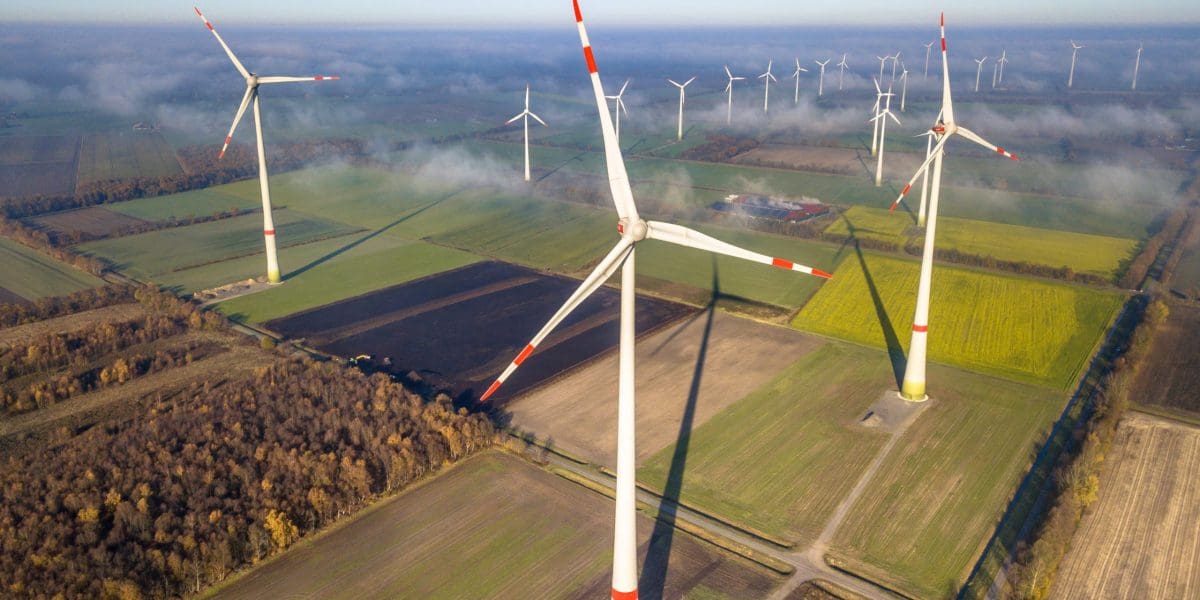The image depicts an aerial view of a wind farm featuring multiple wind turbines spread across a diverse landscape. The turbines, primarily white with distinctive red stripes at the quarter mark and on their three-bladed fans, are set against a backdrop of various fields. These fields consist of green grass, yellow crops, and some barren dirt patches, organized into visible quadrants. To the left, there is a rectangular quadrant of forest trees adding a dark contrast to the scene. A building is situated towards the back of the image, partially obscured by a cloudy haze, which lends a soft focus to that area of the photograph. The foggy conditions, combined with the faint clouds visible on the horizon, give the setting a tranquil, ethereal quality.